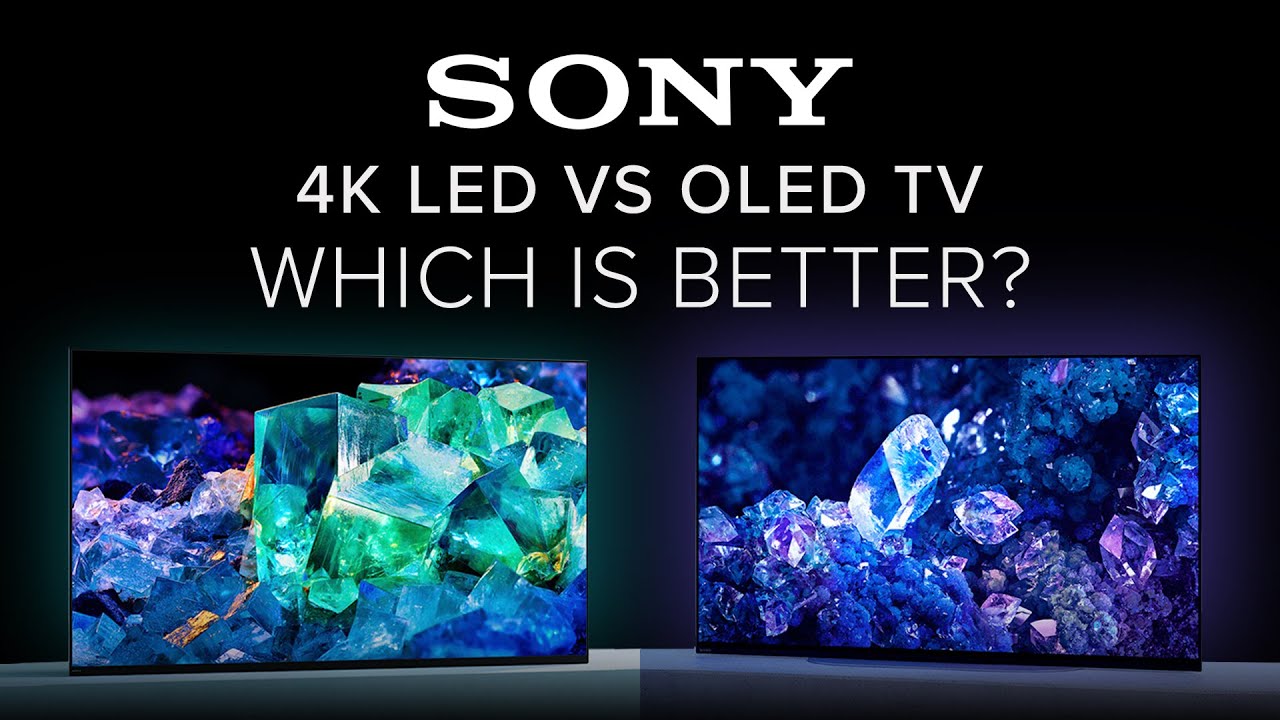The image is a YouTube video thumbnail featuring a display comparison between two Sony televisions under the title "Sony 4K LED vs. OLED TV, which is better?" in white text at the top against a black background. The televisions are positioned side by side on a platform, which is gray on one side and blue on the other. Both TVs have thin, almost borderless black frames and are displaying vibrant images of crystals. The TV on the left showcases a green, turquoise gemstone with several violet and pink crystal formations, while the TV on the right exhibits a more blue-dominant crystal with light white highlights and disorganized purple accents, creating a striking contrast between the two displays.